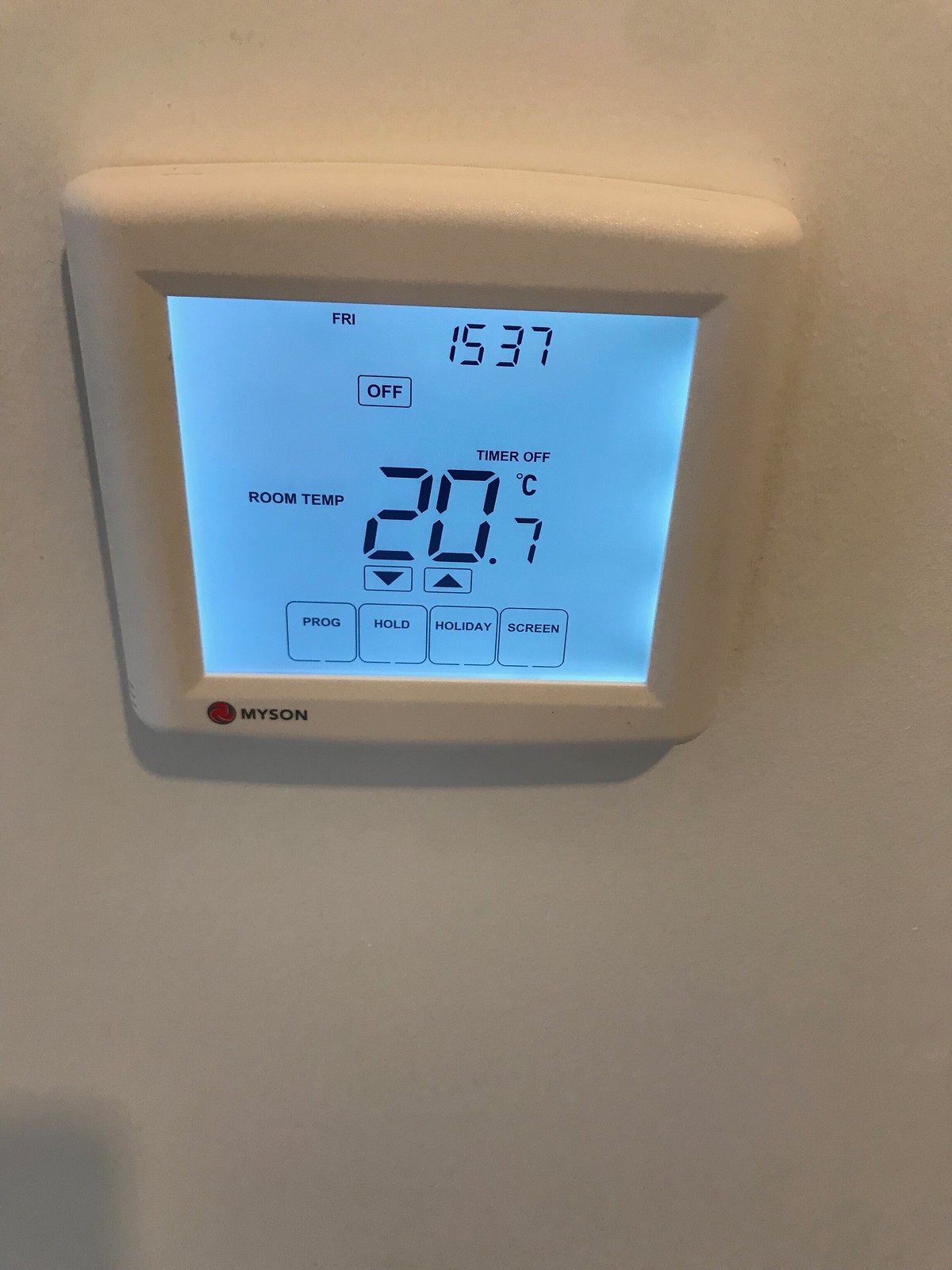This photograph features a Meissen thermostat installed on a pristine white wall, enclosed in a sleek white casing. The device boasts a light blue digital display with crisp, black text. Prominently displayed at the top of the screen is "FRI" for Friday, followed by the time "15:37," indicating it is 3:37 PM. Below the time, the thermostat reads "OFF," encased in a small box, signifying that the heating or cooling system is not currently active. The room temperature is prominently displayed as "20.7°C," with "TIMER OFF" positioned just above it. 

Flanking the temperature readout are two small blackout boxes, each containing an up and a down arrow, presumably for manual temperature adjustments. At the bottom of the screen, there is a row of four menu options, each labeled in bold, capital letters: "PROG" for program, "HOLD," "HOLIDAY," and "SCREEN." These menu options are clearly delineated with dark black text against the light blue backdrop, ensuring easy visibility.

Adjacent to the thermostat, the word "MYSOH" is printed in black text, with the Meissen logo—a black circle containing red stylized motifs—located next to the brand name. This combination enhances the aesthetic appeal of the otherwise functional device, blending modern technology with elegant design.